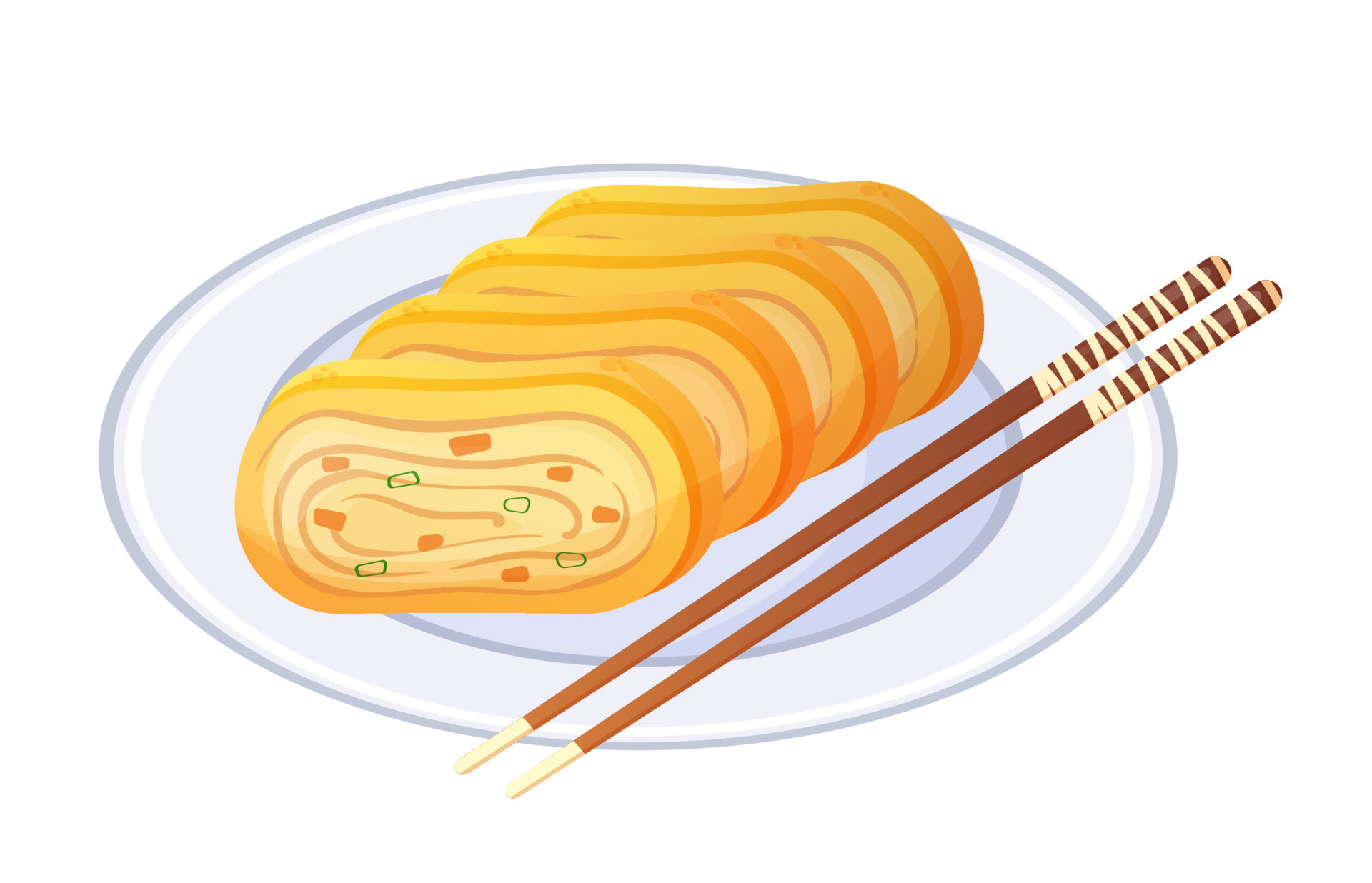This illustration depicts a cartoonish meal set against a completely white background. Central to the image is a white plate with subtle light blue shading, which holds four oblong pieces of food resembling a sliced omelette or a rolled cake. Each slice is a vibrant yellow to orange color with varying shades, showcasing a swirly interior with light brown, light yellow folds and embedded chunks that appear to be green onions and possibly meat. To the right of the plate, a pair of brown chopsticks with white tips and a white string wrapped around their upper ends are laid diagonally across, adding a touch of detail to the scene. The image, rendered in a digital or AI-generated cartoon style, emphasizes a blend of detailed textures and colors, presenting a visually appealing depiction of an imaginative meal.